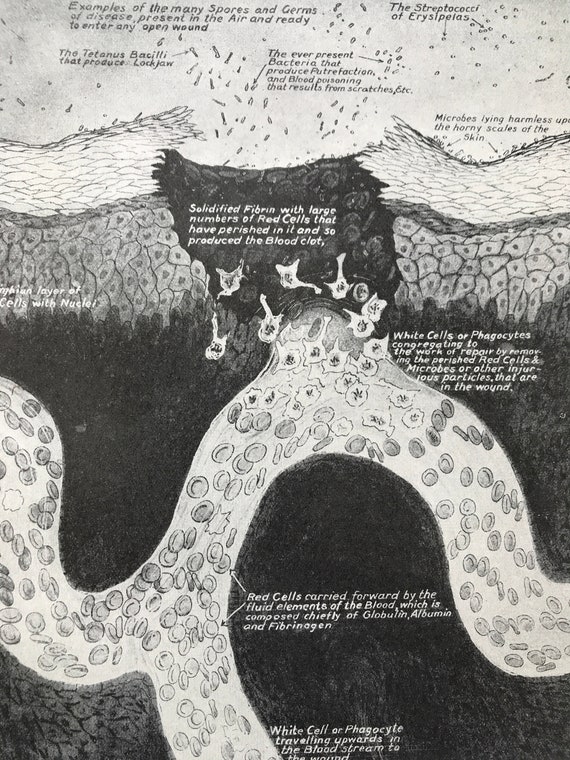This is a detailed black-and-white hand-drawn diagram illustrating the process by which germs, spores, and bacteria infiltrate the skin through an open wound and enter the bloodstream. The upper part of the image features drawings of microscopic creatures, with text and arrows identifying them, such as the streptococci of erysipelas and tetanus bacilli associated with blood poisoning and lockjaw. The text reads, "Examples of the many spores and germs of disease present in the air and ready to enter any open wound."

As the eye moves downward, the diagram showcases a broken section of skin with a detailed depiction of cellular reactions. The exposed cells beneath the skin are vulnerable to the invading bacteria. White cells or phagocytes are shown congregating at the wound, working to repair the damage by attacking the invading microbes and remanufacturing perished red cells. The image also details a blood clot composed of solidified fibrin and numerous red cells, indicating the body's natural defense mechanisms. 

Text and arrows further elucidate the various components, explaining the roles of red cells carried by the fluid elements of the blood—chiefly globulin, albumin, and fibrinogen—in combating the infection. Overall, the diagram meticulously explains the complex interactions between the invading germs and the body’s cellular defenses, providing an educational overview of the infection process and immune response.